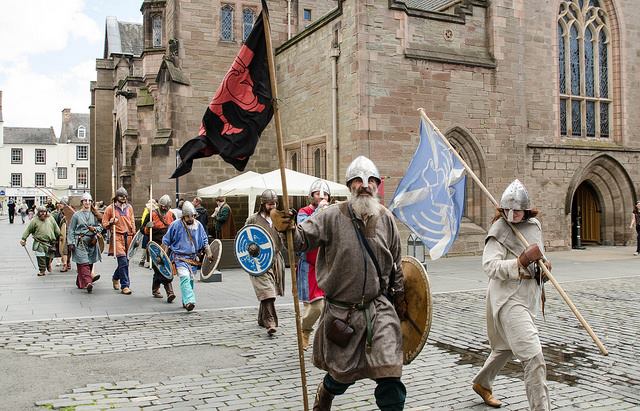This horizontal rectangular photograph captures a vibrant medieval reenactment set against the backdrop of a grand, medieval European church, sprawling as large as a city block. The church, characterized by its impressive arched doors, large windows, and intricate brickwork, stands majestically in the background, contrasting with the house-like buildings seen further away. The scene is bustling with re-enactors, some seemingly Viking-themed, who are assembled in a long, orderly column. 

In the foreground walks a distinguished, older bearded man in a gray tunic with long white hair and a white beard, his head adorned with a helmet featuring a nasal guard. He is equipped with a sword or spear in one hand and a shield in the other. Beside him is a smaller figure, a woman in white, also wearing a nasal helmet and carrying a flag. She mirrors his stride, adding a synchronized grace to their march. The flags billow in the wind; one displays a vivid blue bird, while the other shows a darker design with a red emblem, partially obscured.

The column of re-enactors trails behind them, populated with individuals, possibly all men, dressed in early medieval attire such as tunics and underskirts, all carrying shields and flags as they transition from the plaza around the church to a cobblestone street, immersing the viewer in a vividly historic and highly detailed tableau.